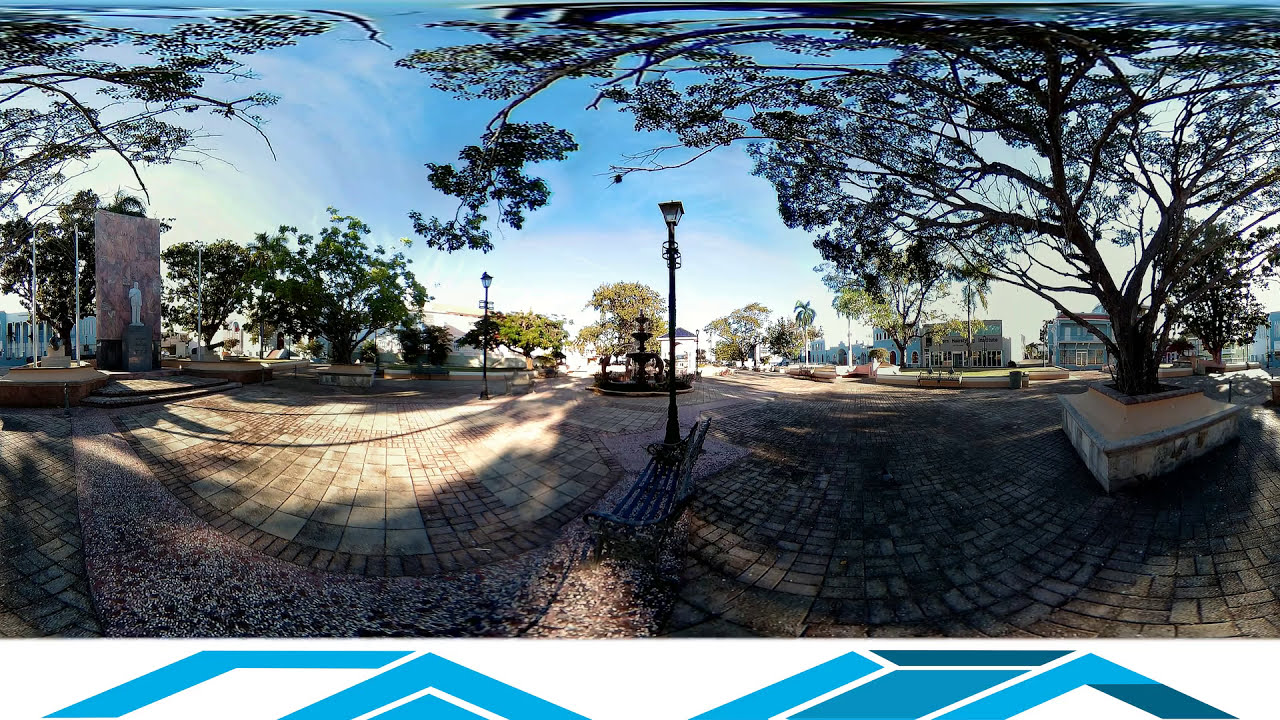The image captures a panoramic view of a tranquil outdoor park, seemingly set within an academic or residential area, influenced by the clear blue sky and bright afternoon sunlight. Dominating the foreground, a semicircular path of pavers frames the scene, with two distinct sections on either side. To the right, a tree emerges from a square pedestal set among the pavers. The left side features a step leading up to a prominent white statue, positioned against a granite wall, possibly indicating a tribute or monument area. Behind the statue, several flags can be seen, adding to the solemn ambiance.

Central to the image stands a lamppost, casting its light over the pavers, while other lampposts and park benches complement the serene atmosphere. Further to the right, the scene reveals two or three homes with varying hues of blue and white, contributing to the area's residential feel. The presence of smaller buildings here suggests a campus-like environment, potentially housing classrooms.

In the background, amidst open sunlit spaces, numerous trees and paved roads trail into the distance, enhancing the picturesque setting. Despite the absence of people, the park emanates a sense of quiet repose. At the very bottom of the photo, a separate section features symbolic blue graphs, distinct from the main image. This intricate portrayal of the park effectively combines natural beauty, architectural elements, and a solemn monument area, encapsulating a peaceful, well-maintained public space.